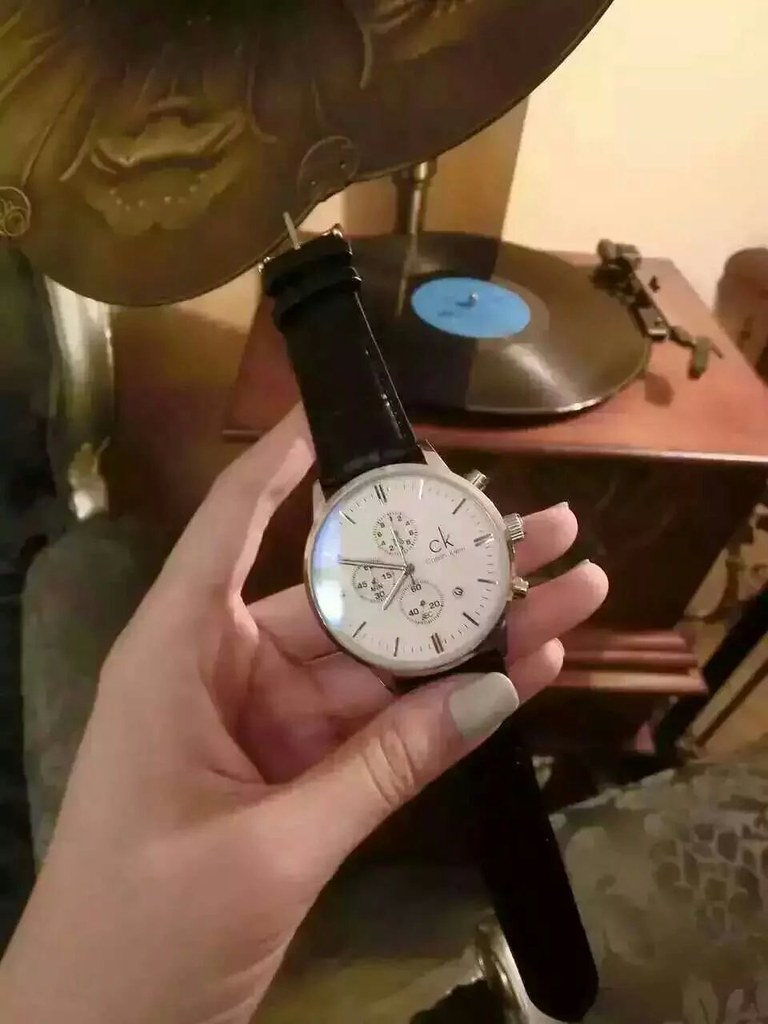In this close-up photograph, a person with light gray or white manicured nails, and light complexion, holds a large Calvin Klein watch set to just before 8 o'clock. The watch has a black leather strap with silver around the outer edge of the white face, which features the black CK logo and Calvin Klein branding. The watch face has Roman numerals for the hours and hash lines for the minutes, with silver hour and minute hands, and three smaller dials within the main face. This intricate watch is possibly a men's design, distinguished by its black leather band and detailed dials showing intervals of 60, 40, 20, and smaller increments. In the background, the room appears to be a living area with beige or cream-colored walls and light brown carpeting. Dominating the backdrop is a wooden antique record player with a large, ornate brass horn and a black record spinning at its center, highlighted by a dark blue circle. The record player rests on two-tiered maroon-brown legs, adding a vintage charm to the cozy and elegant setting.